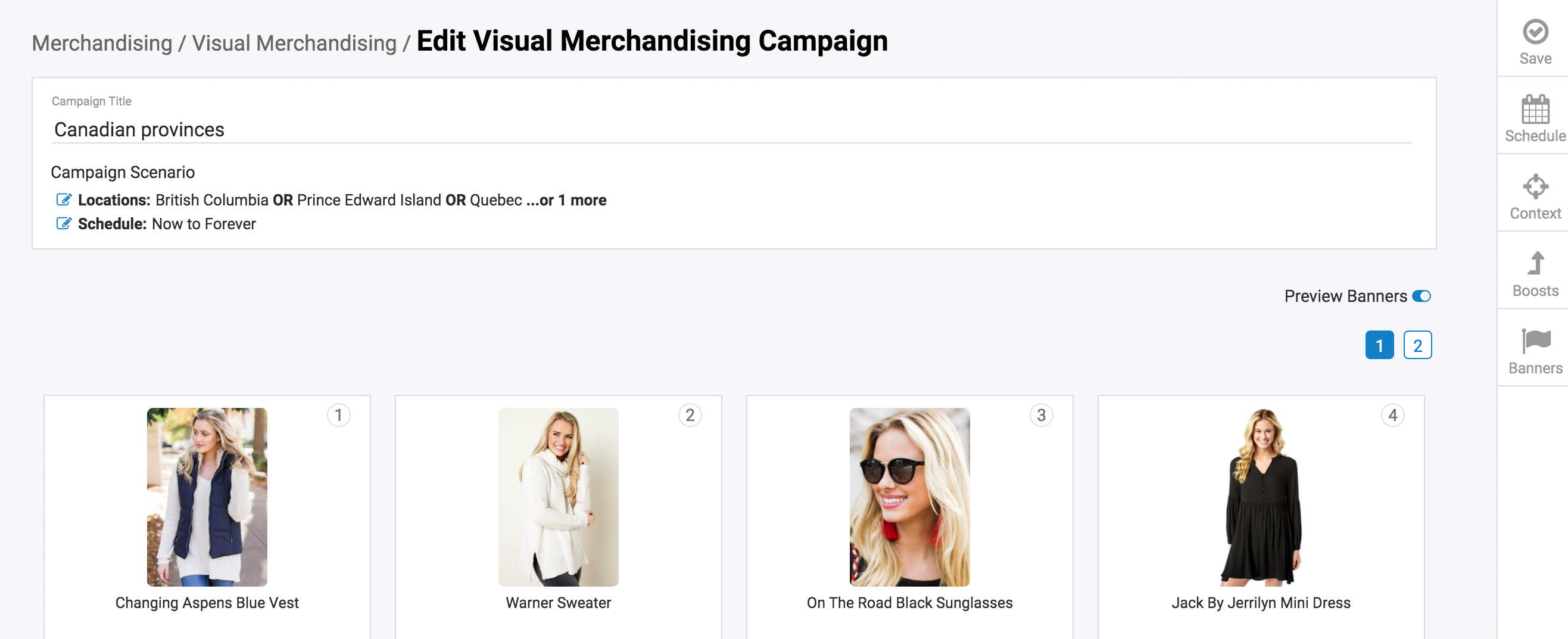The web page displayed is dedicated to a visual merchandising campaign, featuring a minimalist design with a grayish background. On the top left, there’s a breadcrumb navigation trail indicating the current location within the site as follows: Merchandising > Visual Merchandising > Edit Visual Merchandising Campaign.

The central focus of the page is a merchandising campaign titled "Canadian Provinces." Directly beneath the campaign title, there’s a section labeled "Campaign Scenario" detailing various locations: British Columbia, Prince Edward Island, and Quebec, with the campaign scheduled to run indefinitely.

Beneath the campaign scenario, there are four numbered images showcasing a blonde woman modeling different items. The first image is captioned "Changing Aspen's Blue Vest," featuring the woman wearing the vest. The second image is labeled "Warner Sweater," depicting her in the said sweater. The third shows her in "On the Road Black Sunglasses," and the fourth image is titled "Check by Jerilyn Minidress," showing her in a black minidress.

On the right side of the page, there is a vertical array of functional buttons including "Save" (with a check mark), "Schedule," "Contacts," "Boost," and "Banners," allowing users to manage various aspects of the campaign.